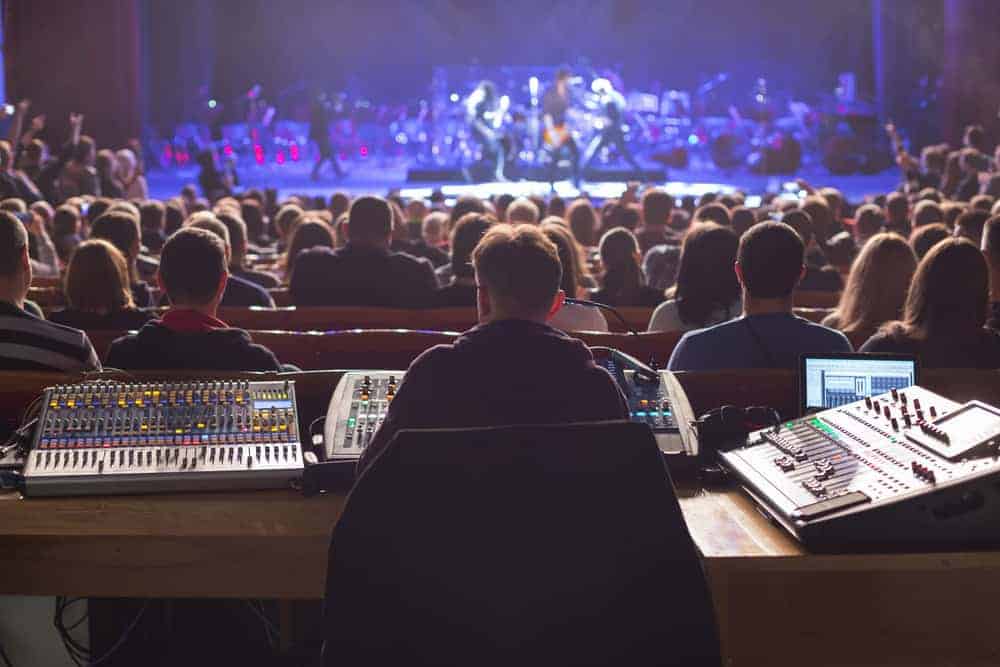The image depicts a rock band performing on stage in a theater-like setting, illuminated predominantly by purple stage lights. In the forefront, a man sits at a mixing board, meticulously adjusting volumes and possibly recording the performance. A diverse crowd of fans, seated in several rows, watches the band intently. The band's frontman wields a guitar, accompanied by additional guitarists and a drum kit positioned at the back of the stage. The scene features a color palette of dark blue, purple, red, brown, black, white, and silver, adding to the vibrant yet intimate atmosphere of the concert. The meticulous sound production and the audience's focused engagement emphasize the event's immersive experience.